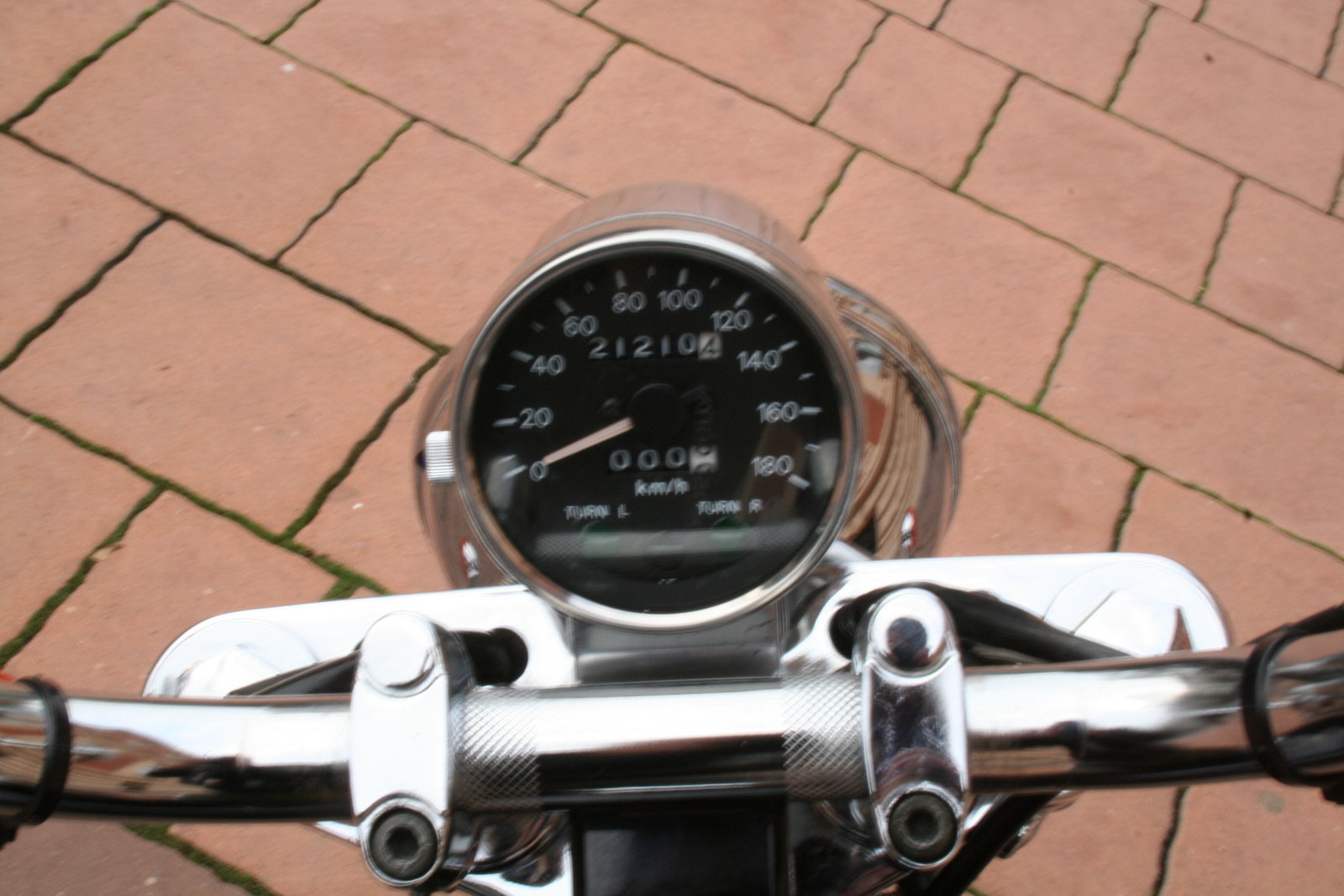In this evocative outdoor photograph, we are presented with a charming cobblestone street characterized by its terracotta-hued bricks. The cobblestones, irregular in size and featuring wavy edges, display the tell-tale signs of age with patches of moss sprouting between the cracks, adding a sense of rustic allure. Dominating the forefront center of this image, we catch a top-down glimpse of a motorcycle's handlebars. The handlebars gleam with a bright chrome finish, further highlighted by a cylindrical chrome speedometer centrally positioned. The speedometer, with its black face, prominently displays the numbered range from 0 to 180, with the dial hand resting firmly at 0. The odometer shows zeros across the board, suggesting that the motorcycle has yet to traverse any distance. This meticulous composition captures a moment poised and ready for a journey, against the timeless backdrop of the weathered cobblestone street.